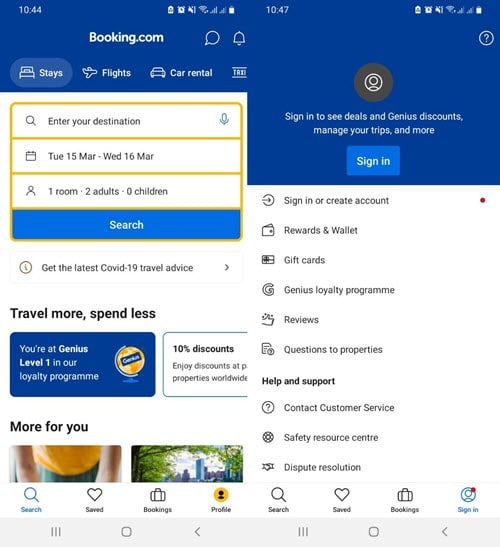This image features two mobile screenshots displayed side by side, both from the Booking.com app.

- **Left Screenshot:**
  - **Header**: At the top, a bold white "Booking.com" logo is set against a blue background. Below this, within the blue header, there are categories labeled: "Stays," "Flights," "Car Rentals," and a partially visible fourth category.
  - **Main Section**: The background is white with three yellow-bordered input fields for: "Enter your destination," "Select dates," and "Number of guests." Below these fields, a prominent blue "Search" button is featured.
  - **Additional Information**: There is a pop-up below the search button providing the latest COVID-19 travel advice, accompanied by a right-pointing arrow for more information.

- **Right Screenshot:**
  - **Header**: The top of the screen has a thick blue banner with an account login icon, followed by a prompt: "Sign in to see deals, Genius discounts, manage your trips, and more."
  - **Main Section**: Dominating the center is a large blue "Sign-in" button.
  - **Additional Options**: Below the button, a vertical list of options includes: "Sign in or create account," "Rewards and wallet," "Gift cards," "Genius loyalty program," "Reviews," "Questions to properties," and a "Help and support" section at the bottom.